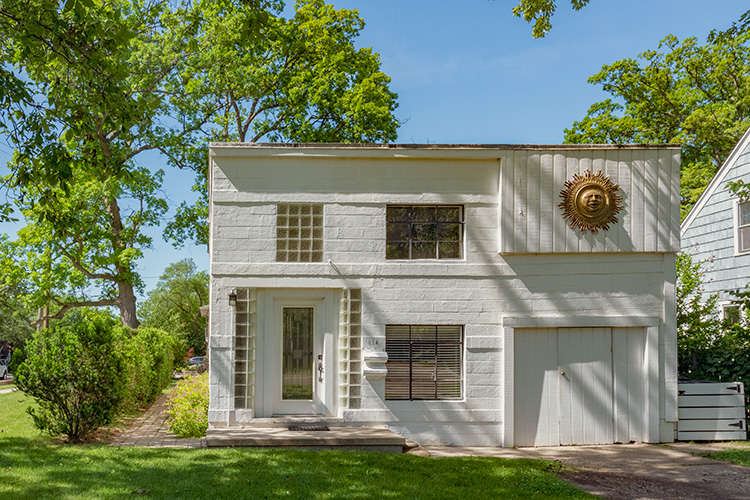The image captures a picturesque white, square-shaped house surrounded by lush greenery under a clear blue sky, indicating it was taken during the daytime. The house is nestled within a neighborhood, encircled by numerous tall, green trees that complement the vibrant grass lawn out front. The house itself is two stories high, with the first floor featuring a door on the left side that has a rectangular patterned window, and a square window in the middle. The upper floor includes two windows, one of which appears frosted. 

To the right side of the house's facade, there’s a decorative golden sun ornament with a human face, adding a touch of charm. A small, white garage with traditional pull-open doors and a narrow driveway are visible. There's also a little white gate leading to a side entrance of the yard, bordered by bushes and a brick walkway on the left side. In the background, the neighboring house, distinguishable by its different siding and triangular shape, peeks into the frame. The overall scene emanates a sense of serene suburban life with its well-kept and timeworn appearance.